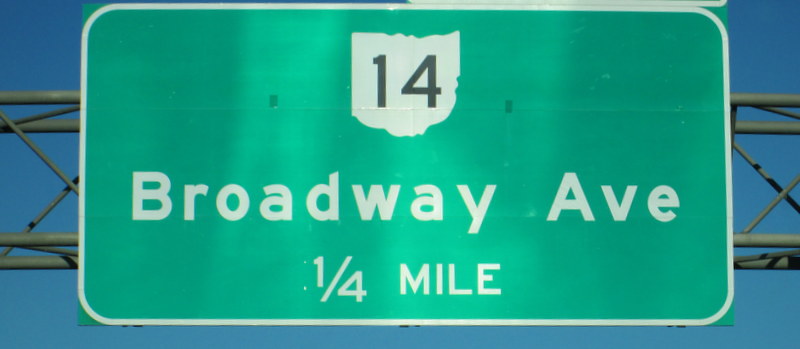The image depicts a large rectangular green highway sign mounted above the road, secured with a series of rusted steel hanger bars. The sign features a white border and prominently displays a white state shape, likely Ohio, with black numbers "14" within it. Beneath this state icon, in bold white letters, are the words "Broadway AVE," and below that, the distance to the turn is indicated as "1/4 MILE" in capitalized white letters. The background showcases a bright, clear blue sky, adding contrast to the green sign. This image appears to be captured from a first-person viewpoint, looking up towards the sign, emphasizing its position above the road.